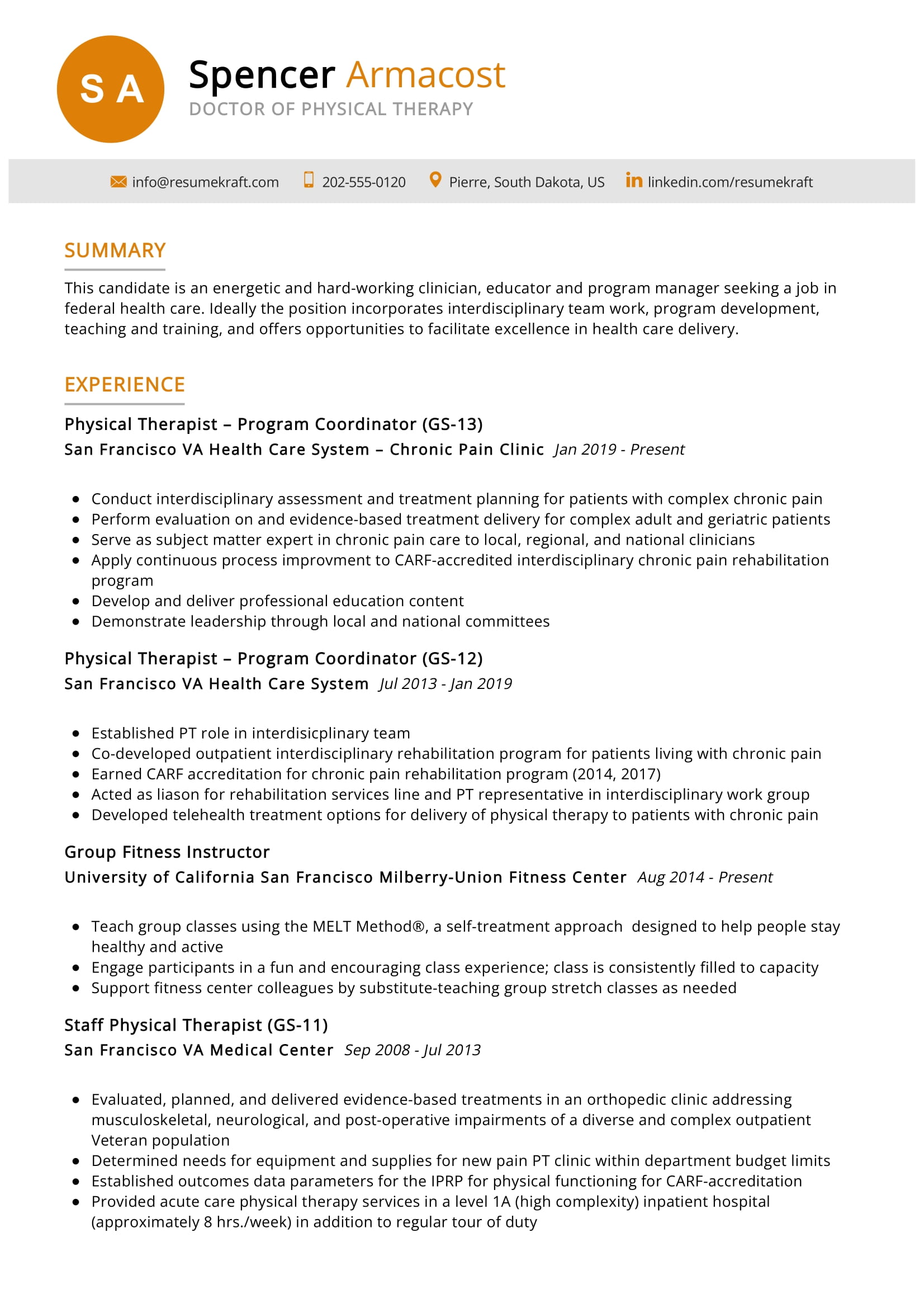The image showcases the resume of Spencer Armacost, Doctor of Physical Therapy. At the top, a yellow circle with the white initials "SA" is present, followed by "Spencer Armacost" with "Doctor of Physical Therapy" beneath it, separated by a gray line running across the page. His contact details, including an email (info@resumedraft.com), phone number (202-555-0120), address (Deer, South Dakota, U.S.), and LinkedIn profile (LinkedIn.com/resume or similar), are displayed in a gray background section.

The content unfolds under an orange "Summary" header followed by a detailed professional history. His roles include:
- **Physical Therapist Program Coordinator (GS-13), Chronic Pain Clinic, San Francisco VA Health Care Center** from June 2019 to the present, 
- **Physical Therapist Program Coordinator (GS-12), San Francisco VA Health Care System** from July 2013 to January 2019,
- **Group Fitness Instructor, University of California, San Francisco, Mulberry Union Fitness Center** from August 2014, and
- **Staff Physical Therapist (GS-11), San Francisco VA Medical Center** from September 2008 to July 2013.

The resume is styled with white and gray backgrounds, and text colors varying from black to gold, structured with central alignment and multiple levels of bullet points detailing his rich professional experience.